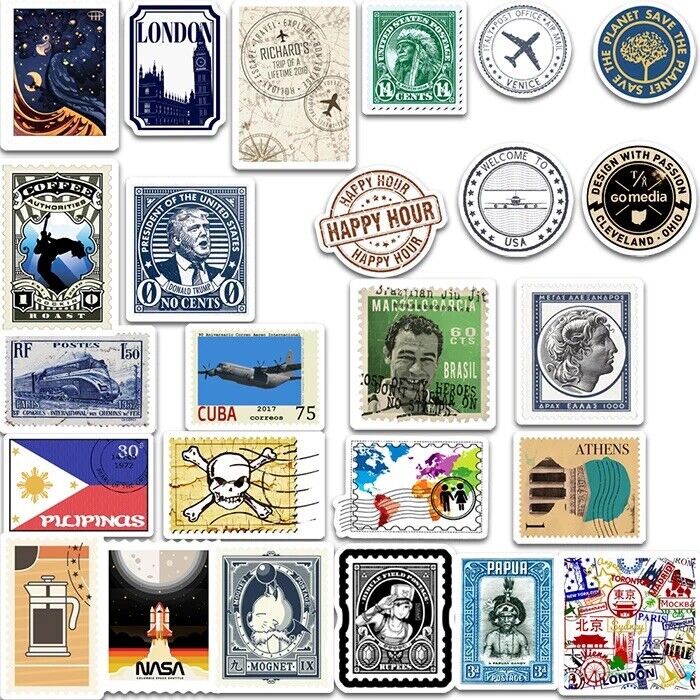The image is a detailed collage of various stamps, possibly mixed with postcards and stickers, all set against a white background. These items are arranged in a dense, overlapping manner, starting from the top right corner and populating down to the bottom left. The collection contains a diverse array of stamps, primarily rectangular, but also including some circular ones which could be stickers or patches. 

Prominent stamps include one with Donald Trump labeled "No Sense," another featuring London with the London Tower, and one with a skull and bones. Other noteworthy stamps feature the text "President of the United States," NASA's space shuttle, a Greek statue, an airplane, and "Happy Hour." Additionally, there are stamps with phrases like "The plant saves the planet," "Design with passion," and "Go Media Cleveland Ohio." The collection's color palette is vibrant, including blue, white, red, yellow, beige, black, gray, light bluish-gray, green, and blue-green hues. Overall, the image presents an eclectic assortment of commemorative and themed stamps, each adding a unique element to the intriguing mosaic.